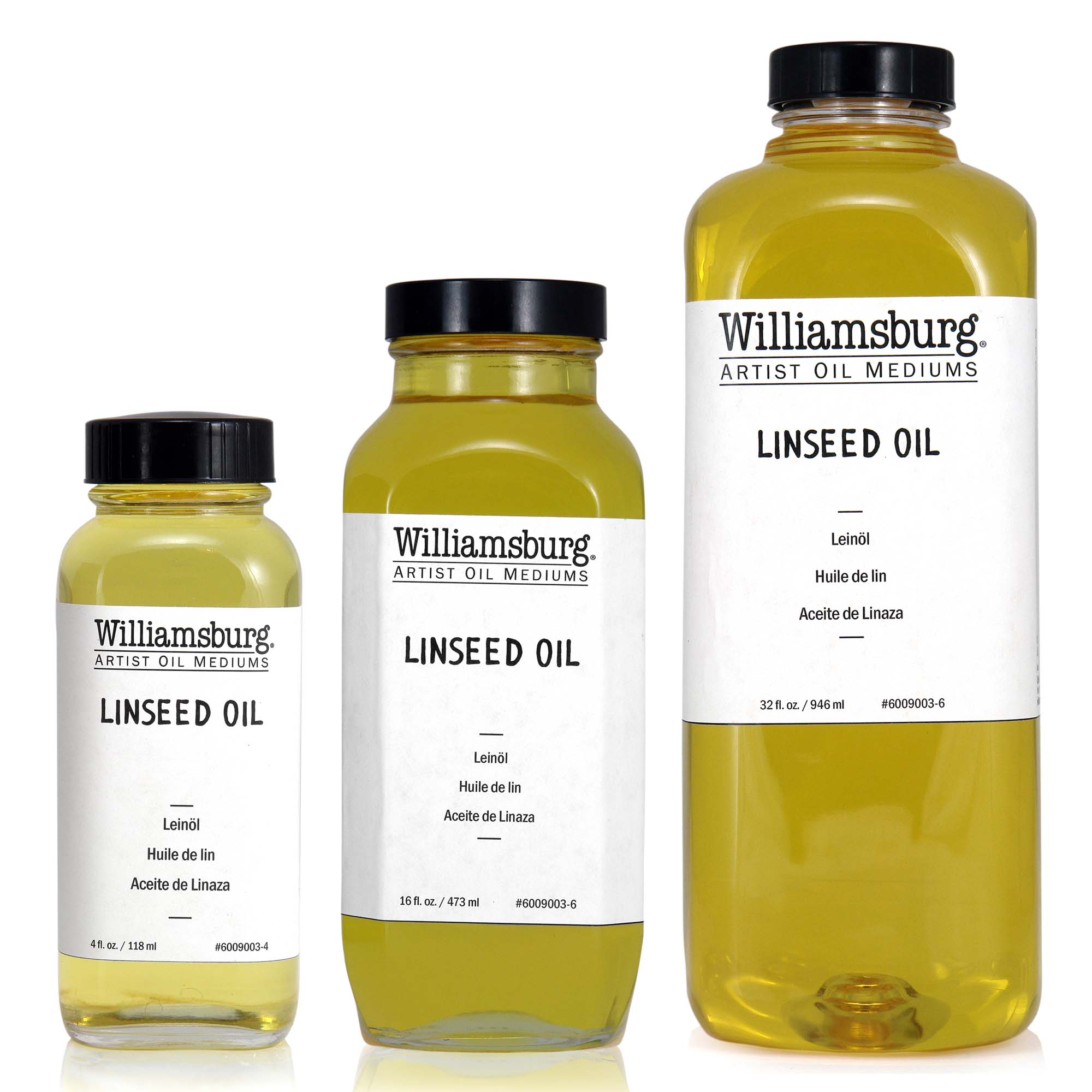This indoor photograph showcases three clear bottles lined up against a white background, each containing a dark yellow liquid labeled as Williamsburg Artist Oil Mediums - Linseed Oil. The bottles, which appear to be made of either plastic or glass, are neatly arranged from right to left in descending order of size: 32 fluid ounces, 16 fluid ounces, and 4 fluid ounces. Each bottle features a white label with black text listing the product details in multiple languages: Williamsburg Artist Oil Mediums, linseed oil, linol, huiledelin, and acetatedelinaza. They all have black screw-on caps, though the cap size on the 16-ounce bottle is disproportionately larger compared to the others. Notably, the 4-ounce bottle appears clearer due to less oil, while the 32-ounce and 16-ounce bottles exhibit a darker yellow hue. The presence of barcodes on the labels further emphasizes the uniformity of the design, except for the variations in bottle size. This image effectively illustrates the different packaging options available for this linseed oil product.